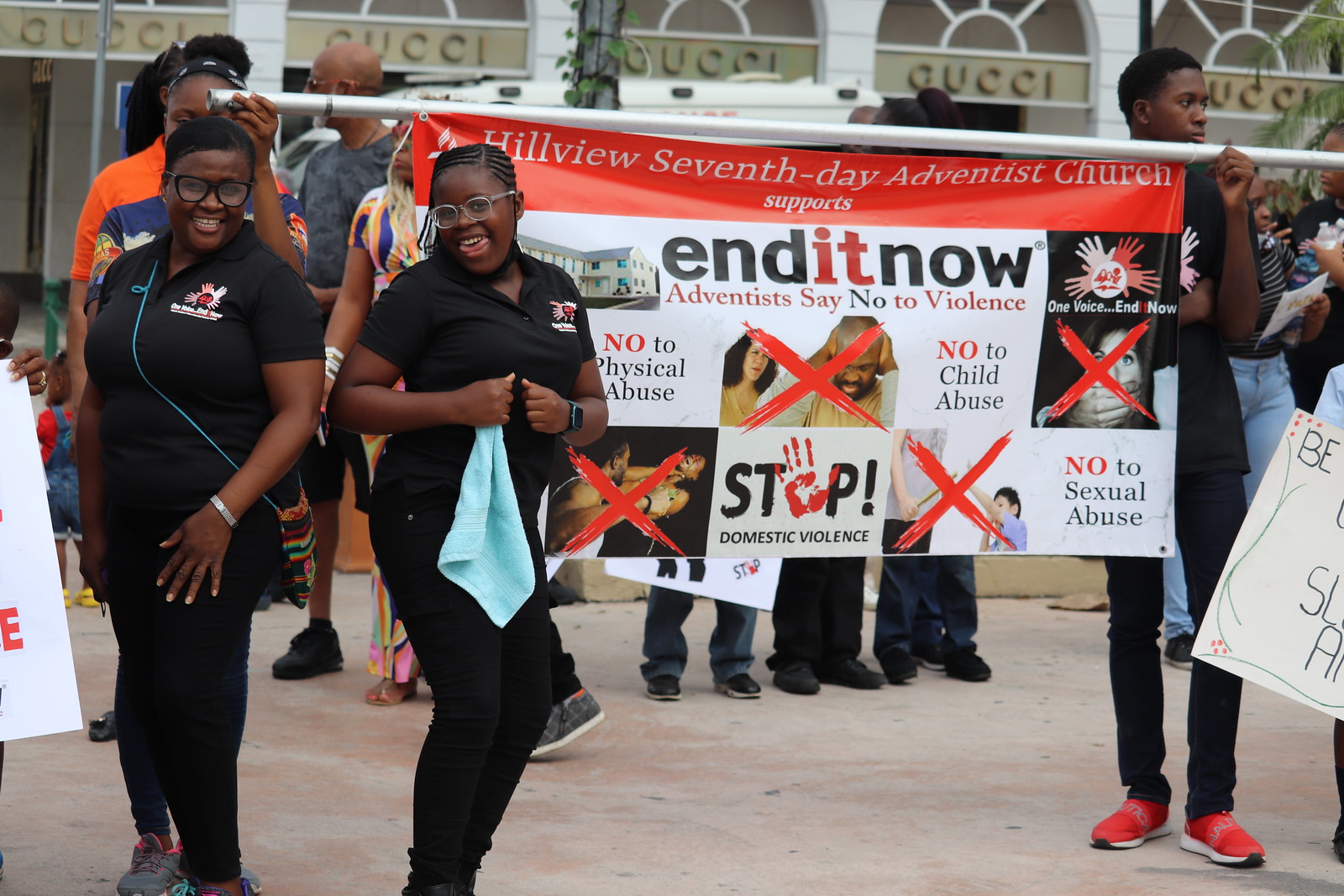This image captures the lively scene of a protest against violence organized by the Hillview Seventh-day Adventist Church. The central focus is on a large canvas banner that reads, in red and white font, "Hillview Seventh Day Adventist Church" with "End It Now" and phrases such as "Adventists Say No to Violence," "No to Physical Abuse," "No to Child Abuse," "No to Sexual Abuse," and "Stop Domestic Violence" in black and red letters. The banner also features graphics depicting acts of violence with big red X marks over them. In the foreground, two African-American women dressed in all-black outfits with matching logos, possibly of the organization, are smiling and striking poses for the camera, wearing glasses and showing a cheerful spirit. Beside them, a young man and another young lady, also dressed in black, hold up the banner with a large metal pole. The woman holding the pole wears an orange top. The protest seems to be taking place on a concrete ground outside a white building with a "Gucci" sign, with cars and more people visible in the background. The overall atmosphere appears joyous and united, as participants stand together advocating for an end to violence.